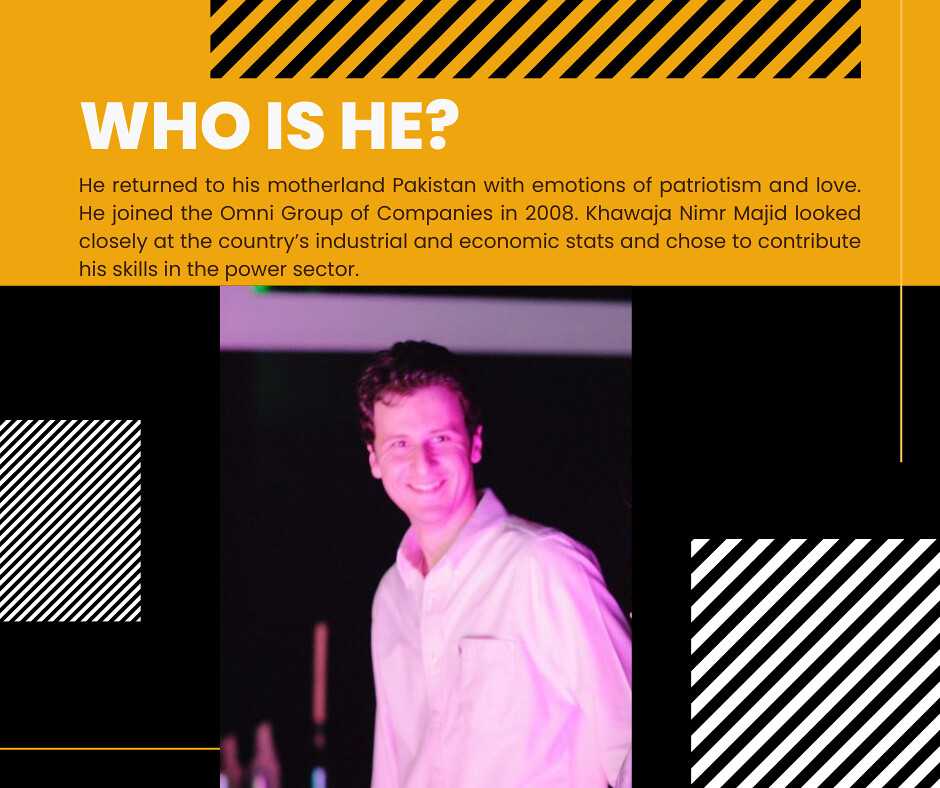The image is an informational graphic split into two primary sections. The top third features a pumpkin-orange background adorned with diagonal black lines that resemble a barcode, spanning from about one-third from the left to nearly the right edge. Beneath these lines, bold white capitalized text reads "WHO IS HE?" with a black font text underneath that states: "He returned to his motherland Pakistan with emotions of patriotism and love. He joined the Omni group of companies in 2008. Khawaja Nimir Majeed looked closely at the country's industrial and economic stats and chose to contribute his skills in the power sector."

The bottom two-thirds of the image has a black background, with a centered picture of a man who has dark, short hair, fair skin, and is smiling. He is wearing a white long-sleeve, button-down shirt with a pocket on the left side. The areas flanking the man's picture feature diagonal and vertical black-and-white stripes, adding a decorative element. These stripes also appear as thicker lines at the very bottom right of the image, balancing the composition.